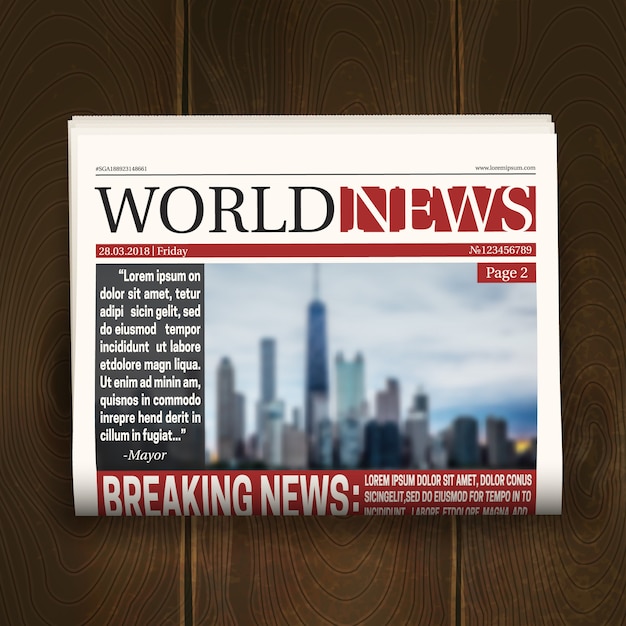A detailed render of a folded newspaper rests on a vertically aligned wooden surface composed of three visible brown planks. The newspaper is centered in the image and appears to be a few pages thick. Across the top of the white newspaper, there is a small black line with fine-print text in the left and right corners that likely includes a website URL. The headline reads "WORLD NEWS" with "WORLD" in large black letters and "NEWS" in large white letters, set against a red background. Below this, a red rectangular band spans the width of the paper, displaying the date "28-03-2018, Friday" on the left and the identifier "number 123456789" on the right. Dominating the right side of the page, a blurry photograph showcases a city skyline under a blue sky with scattered white clouds, labeled "page 2" in white at the top right. To the left of the photo, there is a black vertical band with about ten lines of placeholder text commonly used for display purposes and the word "MAYOR" in white at the bottom. Beneath the photo and slightly to the left, a red section with the heading "Breaking News" displays more placeholder text in white. The detailed elements of the wood and paper textures contribute to the lifelike quality of this render.